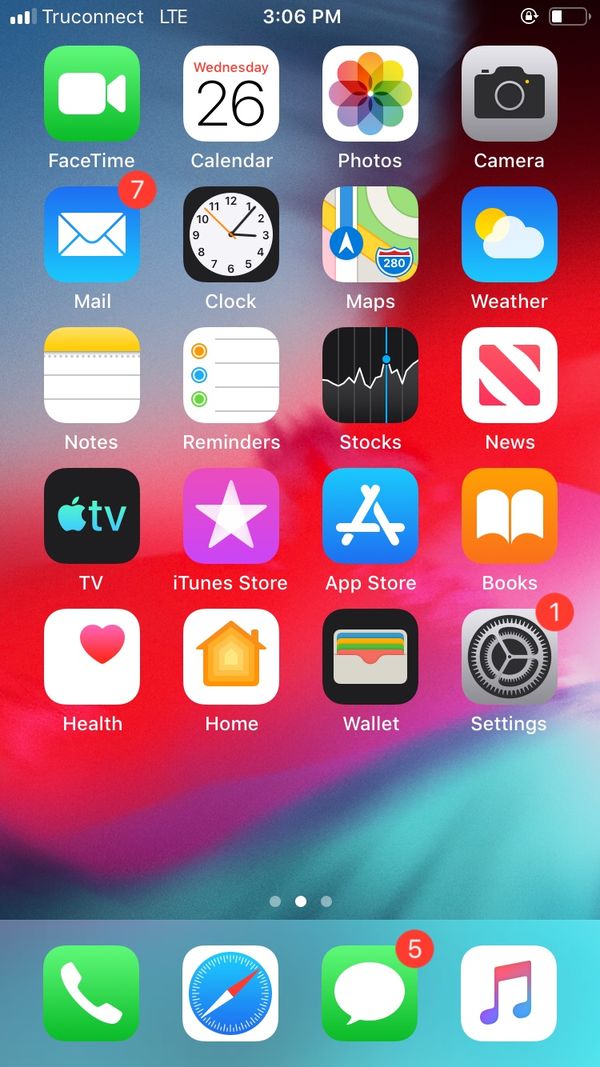### Descriptive Caption for Cell Phone Homepage Screenshot

This vertical rectangular image showcases a cell phone's homepage interface. At the very top, rendered in white font, the display reads "True Connect" followed by "LTE." Centrally positioned is the time, "3:06 PM." To the right-hand side, there's a battery indicator approximately one-third filled, accompanied by a numerical percentage and a small icon.

Moving to the primary section, the screen organizes icons into neatly aligned rows of four apps each, with app names listed below their respective icons.

**First Row:**
1. **FaceTime** - Green icon with a white camera.
2. **Calendar** - White icon displaying "Wednesday" in red and "26" numerically in black.
3. **Photos** - White background featuring multicolored, overlapping flower petals.
4. **Camera** - Light gray background with a black camera icon.

**Second Row:**
1. **Mail** - Blue icon with a white envelope and a red circle with the number 7 in white at the top right.
2. **Clock** - Black icon with a white center showcasing a traditional clock face.
3. **Maps** - Icon depicting a small map design.
4. **Weather** - Blue background with a white cloud and a partially visible sun.

**Third Row:**
1. **Notes** - Icon resembling a notepad with gray lines and a yellow top.
2. **Reminders** - Icon with three colored bullet points and corresponding grey lines.
3. **Stocks** - Black background with graph-like white lines.
4. **News** - White background with a red and white letter "N."

**Fourth Row:**
1. **TV** - Black background with the Apple logo and the word "TV."
2. **iTunes Store** - Purple background with a white star.
3. **App Store** - Turquoise background featuring a stylized "A."
4. **Books** - Yellow-orange background with an open white book.

**Fifth Row:**
1. **Health** - White background with a red heart top right.
2. **Home** - White background featuring an orange house-like icon.
3. **Wallet** - Black background with a multi-colored wallet icon and a red circle at the top right.
4. **Settings** - Gray background with a gear icon and a red circle numbered "1."

At the bottommost section of the screen, there are four additional icons:
1. **Phone** - Green background with a white telephone.
2. **Compass** - White background with a turquoise circle and compass hands.
3. **Messages** - Green background with a white speech bubble.
4. **Music** - White background with musical notes.

The structure and clear organization of the apps and elements provide a comprehensive and user-friendly interface on this cell phone homepage.